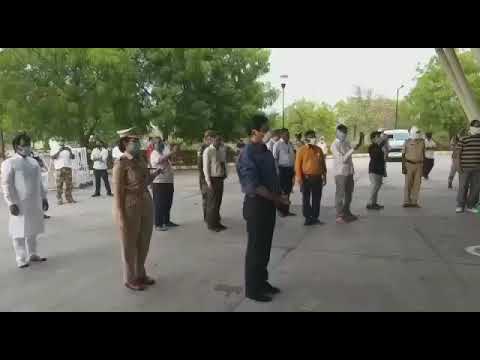The image features a group of people standing in two orderly lines on a rectangular concrete slab with a black border on the top and bottom. The scene is set outdoors under a pavilion, indicated by poles on the upper right corner. The individuals are all wearing masks and facing forward, with several people in each line evenly spaced apart. There appear to be 12 to 17 people in the back line and three in the front, who are dressed more professionally. The attire varies from military uniforms to casual outfits, including a blue shirt and black pants, an orange shirt, and a striped shirt. The background showcases a white sky filled with deciduous trees and a few lampposts, adding a natural scenic element to the setting. All people have their hands by their sides, and the setting is brightly lit by natural daylight.